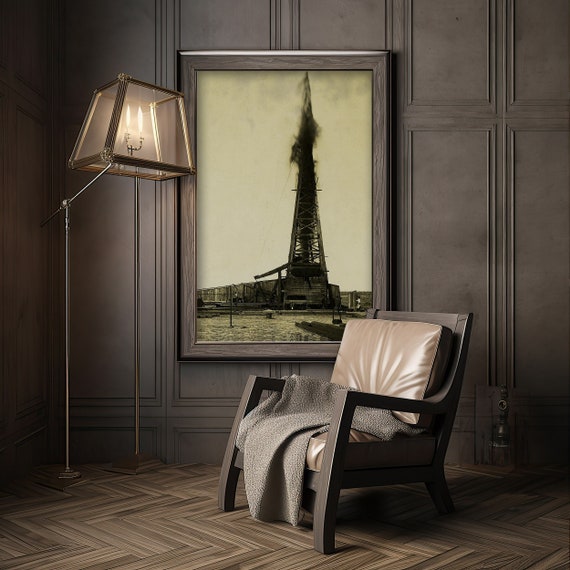The image depicts a warm and cozy room with a predominantly brown color palette, featuring a wooden floor laid out in a chevron pattern with light brown hues. Central to the room is a dark brown Adirondack-style chair adorned with tan leather cushions and a gray wool blanket draped over its armrest. The backdrop reveals brown wooden paneled walls, adding a rustic charm, with a medium-brown wooden framed photograph of an oil derrick striking oil prominently displayed in the center. The left side of the room hosts a unique floor lamp with a thin metal stand and an adjustable swing arm set at a 30-degree angle. The lamp's rhomboid-shaped, bronze-colored glass cover resembles flickering flames, adding to the room's warm ambiance.